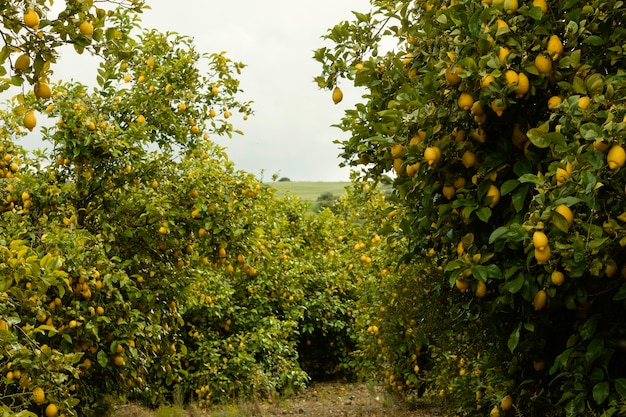This photograph features a lush, well-maintained lemon grove extending across the left, center, and right sections of the image, with lemon trees laden with ripe, yellow fruit. The lemon trees' verdant green leaves provide a striking contrast to the bright lemons, and the grove is segmented by a dirt path running through its center. Scattered on the ground are a few lemons that have fallen. The quaint path creates a natural perspective that draws the viewer's eye forward, flanked by a larger, bush-like lemon tree on the right and smaller lemon bushes on the left. The background opens up into expansive grassy farmland with a subtle rise in the distance, possibly a hill, and the sky above is a hazy gray, devoid of blue and individual clouds. This serene landscape showcases not only the abundance of perfectly ripe lemons but also the tranquil rural setting in which they thrive.